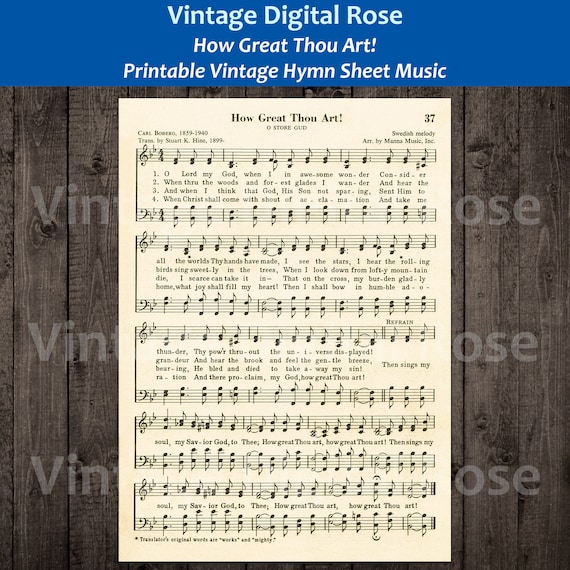This is a detailed advertisement for printable vintage hymn sheet music from Vintage Digital Rose, featuring the beloved hymn "How Great Thou Art." The image prominently displays a blue banner at the top that reads "Vintage Digital Rose, How Great Thou Art, Printable Vintage Hymn Sheet Music." Superimposed text repeating "VIN" on the left and "OZE" on the right suggests the full name "Vintage Digital Rose."

Beneath this banner lies the showcased hymn sheet, marked as page 37, which implies there are at least 37 hymns available for purchase. The sheet music exudes an old-fashioned charm, enhancing its vintage appeal. It features all four verses and the chorus of "How Great Thou Art," accompanied by musical notes and lyrics such as: "Oh Lord my God, when I in awesome wonder, consider all the works thy hands have made; I see the stars, I hear the rolling thunder, thy power throughout the universe displayed. Then sings my soul, my Savior God, to thee; how great thou art, how great thou art."

This product is a meticulously crafted item that vintage music and hymn enthusiasts can print and enjoy, beautifully preserving a piece of musical heritage.